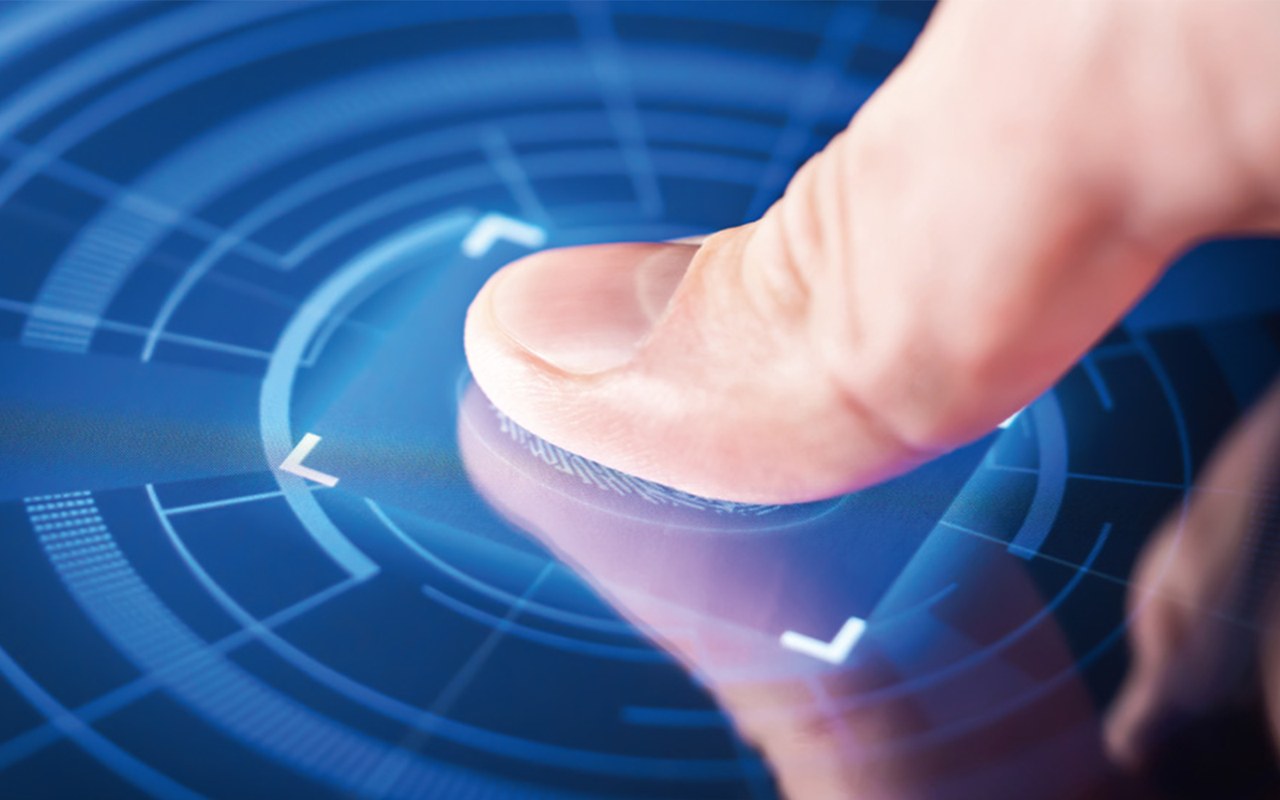The image depicts a highly detailed close-up of a thumb, which appears to be pressing onto a futuristic fingerprint scanner. The thumb is positioned against a computer-like interface that features a thumbprint recognition area, demarcated by a blue square with white notches in each corner. Surrounding this square are concentric circles, resembling a target, set against a reflective, bluish background. The pattern of the thumbprint is visible underneath the thumb, and you can see the undulations of the fingerprint quite clearly. The person using the scanner has light skin with a short, rounded fingernail and a lighter-colored cuticle. The surface of the scanner is glossy, emphasizing the high-tech feel of the device. The image might be a promotional or stock photo, given its polished and almost cinematic quality, reminiscent of technology seen in spy films. The overall aesthetic is very sleek, blue-toned, and reflective, highlighting both the precision and modernity of the fingerprint scanning technology.